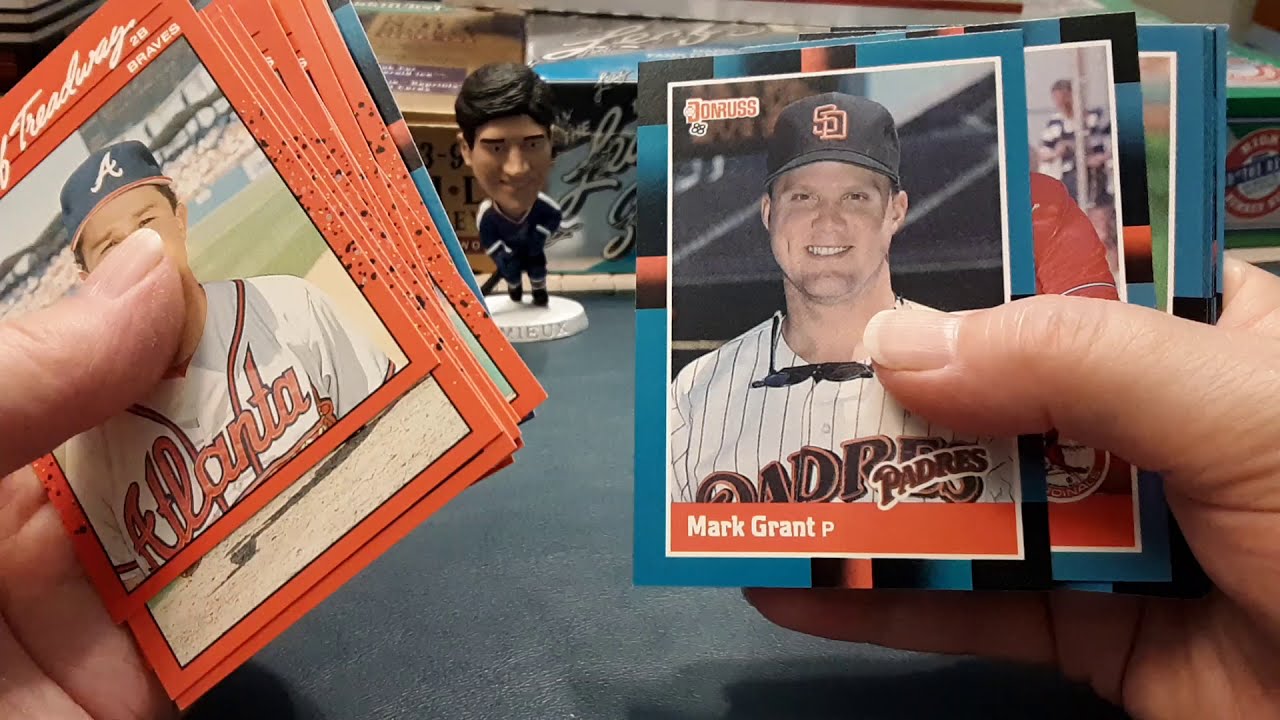In this first-person point-of-view photograph, a person is holding two stacks of vintage baseball cards over a black table. In the left hand, they grip a thick stack of cards, primarily framed in orange, featuring a player from the Atlanta Braves. In the right hand, they hold another stack, notably framed in light blue with black and orange details, with the front card showcasing Mark Grant, a former pitcher for the San Diego Padres, indicated by the name "Mark Grant" in a white font within an orange box at the bottom of the card. Positioned centrally between the two hands is a bobblehead figurine, depicting a player with short brown hair dressed in a blue jersey and pants adorned with white stripes, resting on a white base. Behind this focal point, the background reveals indistinct boxes likely containing more baseball cards and shelves, suggesting the setting might be a collectibles store.